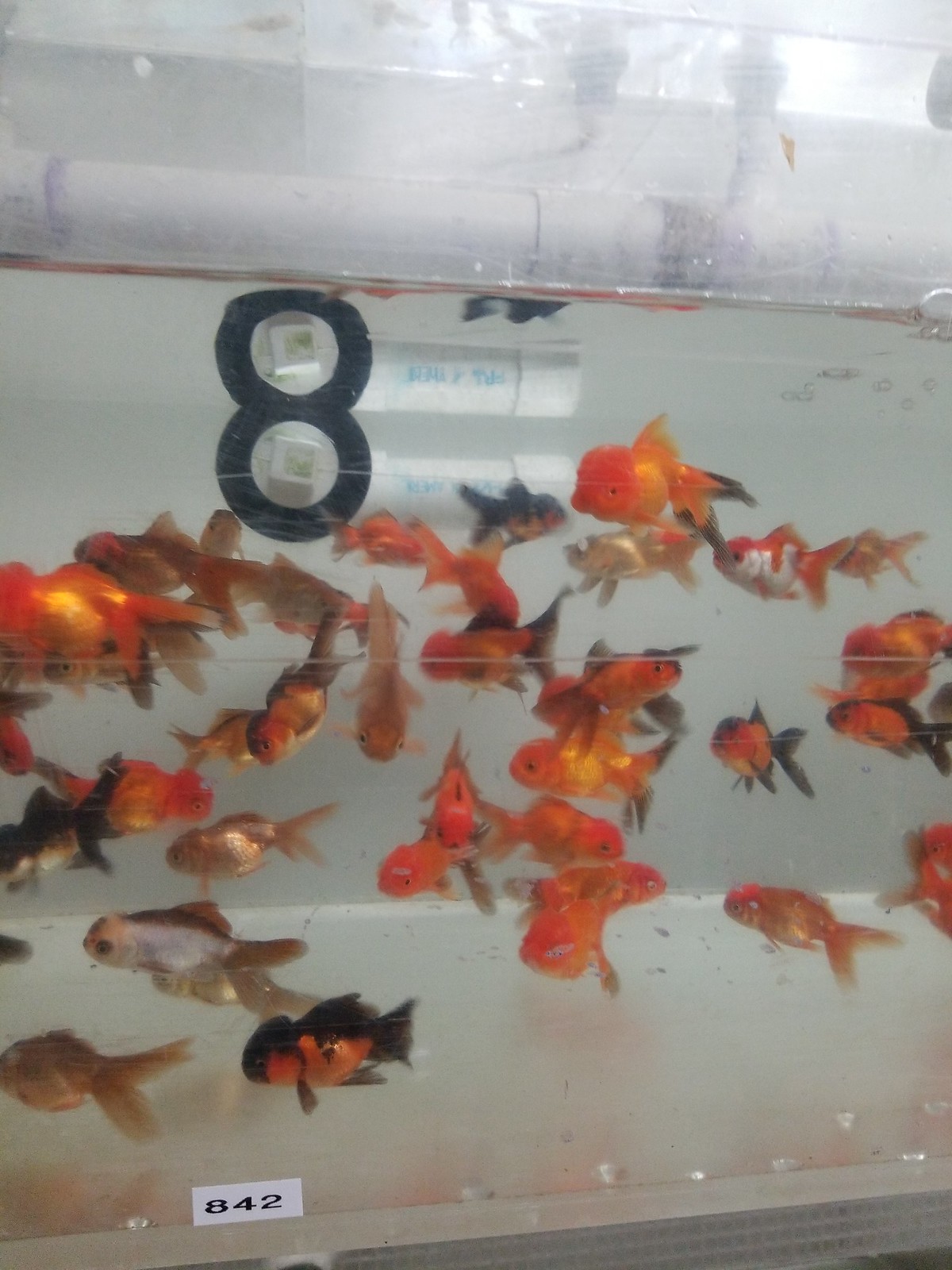The image features a side view of a large, uniquely-shaped fish tank, likely part of a research setting. The tank has a distinct cylindrical-quarter shape, with a prominent black number '8' on the left side just below the water line and a sticker at the bottom that reads '842' for identification. The water inside is somewhat dirty and cloudy, with algae floating on top. There are approximately 25 to 30 small fish, mainly orange goldfish, swimming in various directions. Some fish exhibit different colorations, including silver and black-orange combinations. At the top of the tank, a large white tube spans from left to right, visible despite the blurry and dirty tank walls. The background shows a grayish wall and a slim window on the top right with light streaming through. Two smaller pieces of PVC pipe are also visible at the back of the tank.